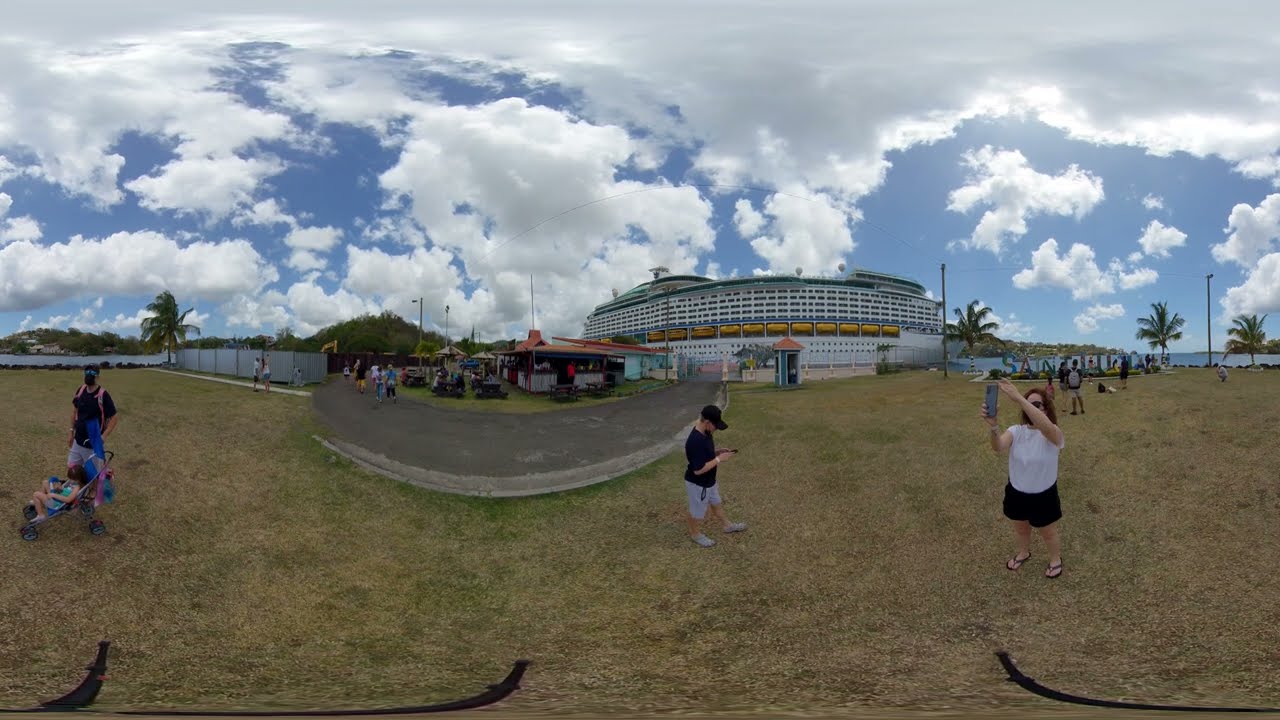In this picturesque outdoor scene, several people are gathered on a predominantly brown and beige grassy field speckled with patches of green. The field is visibly weathered, with a starkly contrasting gray, upside-down rainbow-shaped paved path cutting through the middle. Clustered towards the left side of the image, small groups of people stroll under a bright blue sky adorned with large, white clouds.

Dominating the center of the scene is a large, white, multi-story building that resembles a cruise ship, complete with numerous windows and yellow lifeboats. There is a white fence and colorful signage at the bottom of the building that appears to spell out "San Diego," adding a splash of vibrancy to the otherwise muted tones of the grass and pavement.

In the foreground, a woman in a white T-shirt and black shorts holds a cell phone for a photo, while nearby, a man in a black shirt, black cap, and gray shorts is focused on his phone. To the left, another man, donned in a mask, stands with a child in a baby carriage. Scattered throughout the field are various other people, some seated at umbrella-covered tables and others walking along the paved path.

Four tall palm trees rise against the horizon, adding to the scenic vista, and the overall impression is one of a pleasant, sunny day, likely in a park or recreational area. The sky, with its beautiful interplay of clouds and light, dominates the upper half of the image, suggesting an enjoyable day spent outdoors.